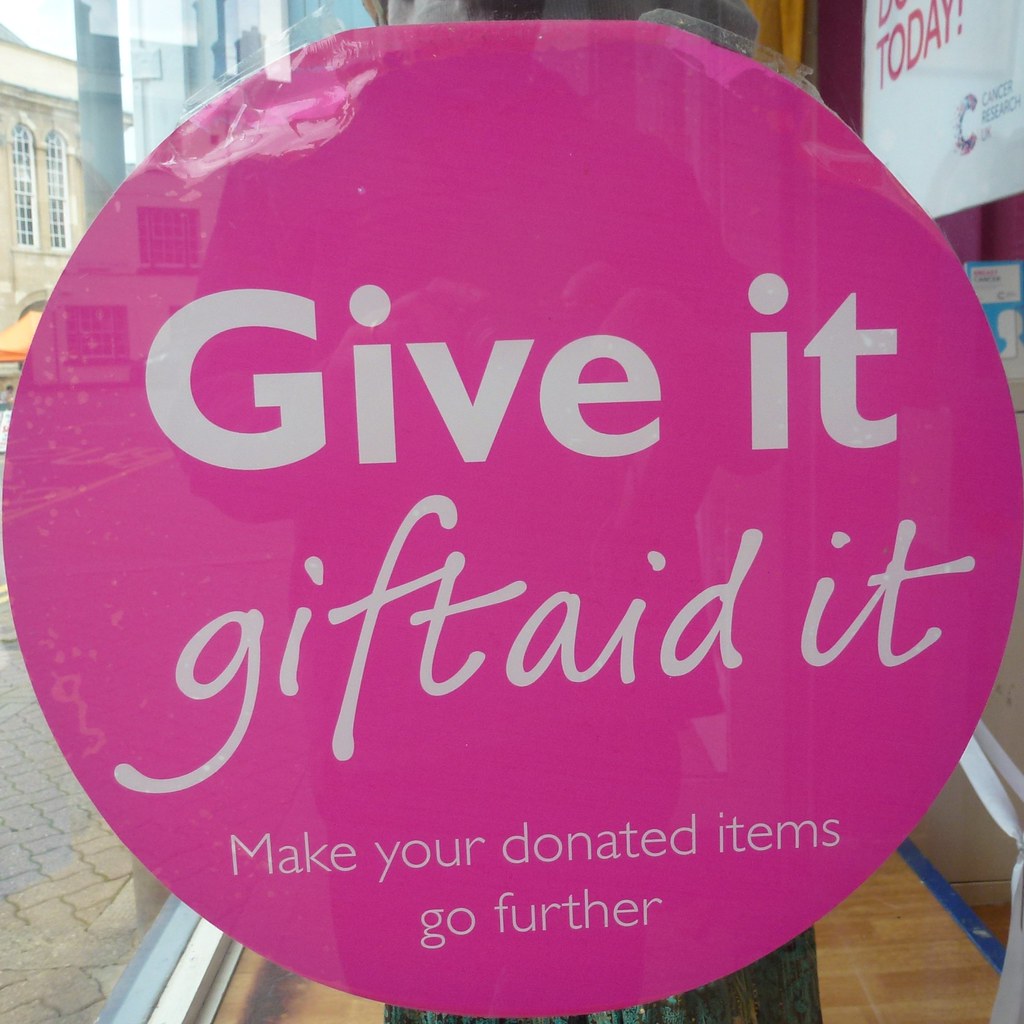The photograph captures a scene through a window, with the photographer's hands and camera faintly visible in the glass reflection. At the center of the window is a large, circular pink sign with slightly peeling edges, secured with scotch tape. The sign features white text: at the top in a sans-serif font it reads, "Give it," followed by "Gift Aid It" in a cursive handwriting font, and at the bottom in small sans-serif font, it states, "Make your donated items go further." In the background, outside the window, there is a majestic cathedral-like building with large arch grid windows, situated amidst a cobblestone road or paved concrete bricks. Inside the windowed area, there is a hardwood floor and a white sign with red capital letters that says "TODAY."